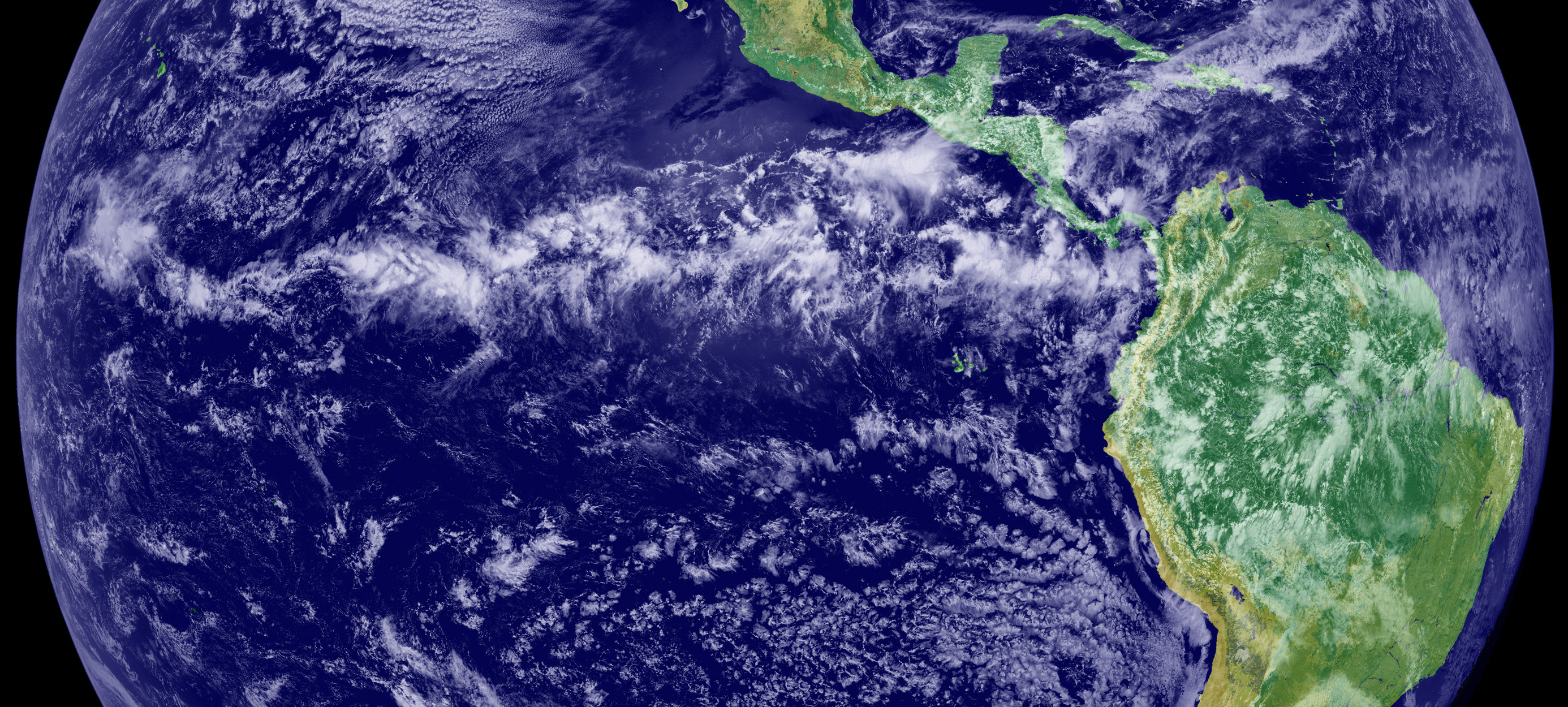This rectangular, landscape-oriented image captures a partial view of Earth, with the top and bottom cut off, leaving the middle section visible. Dominated by the deep blue of the oceans, the Earth's surface is interspersed with wisps of white clouds, hinting at weather patterns. Towards the center and lower right, the geographical features of Central America, Mexico, and the upper part of South America are recognizable, with the landmasses portrayed in shades of green and touches of yellow. To the upper left, the black expanse of space envelops the scene, accentuating the planet's curvature. Off the coast of Central America, some details of the Caribbean islands are also discernible. This image effectively places emphasis on Earth's vibrant waters and dynamic atmosphere amidst the vast, dark void of space.